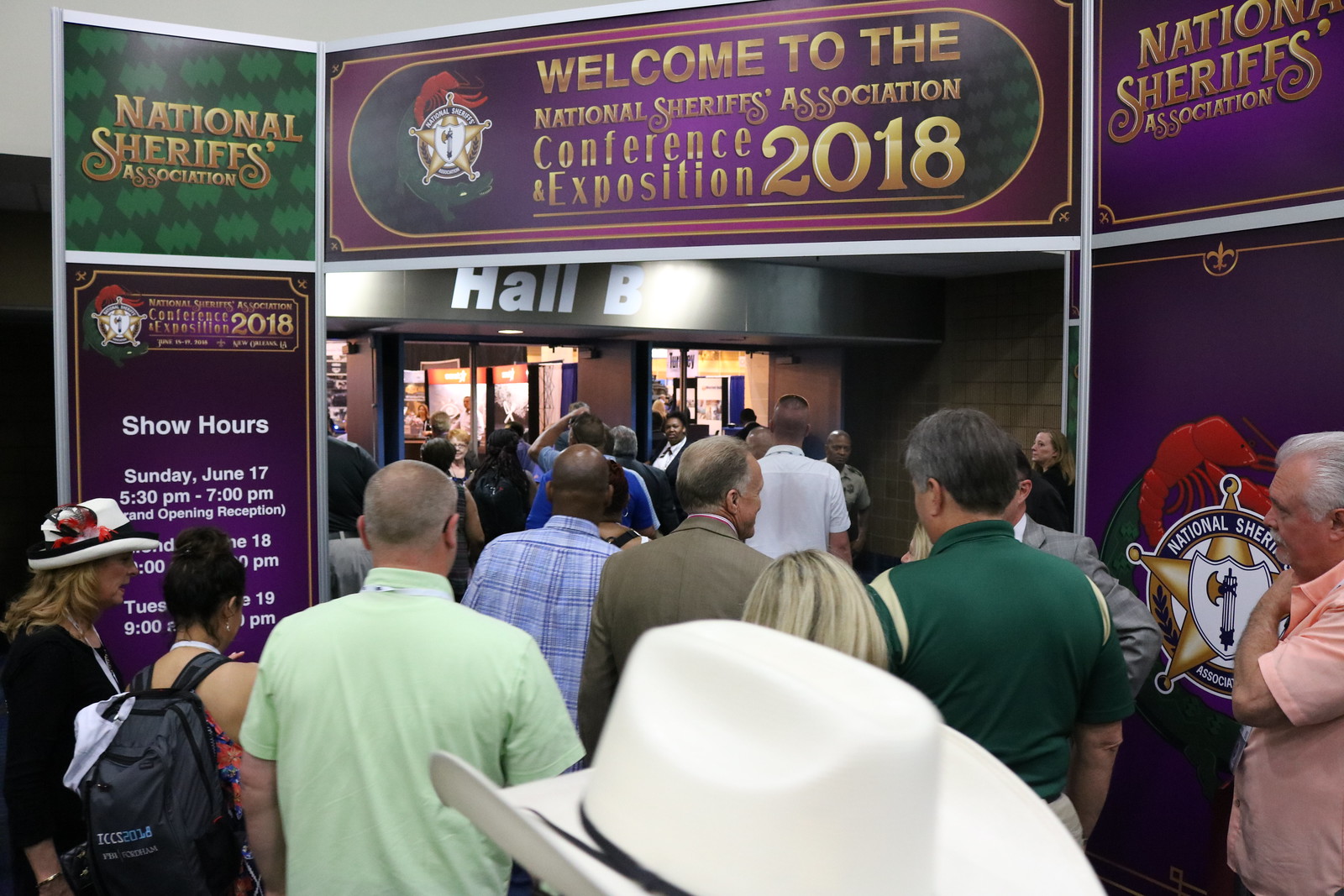The image depicts a bustling booth at the National Sheriff's Association Conference and Exposition 2018, held in New Orleans, Louisiana. The entrance is framed by three visible walls with prominent signage welcoming attendees. Above the entryway, a large banner reads "Welcome to the National Sheriff's Association Conference and Exposition 2018," with "2018" presented in a large, eye-catching font. To the left of the banner, a green section states "National Sheriff's Association," while the right side is adorned with purple, repeating the same message.

In the foreground, a detailed sheriff's badge with a red background stands out, accompanied by a visible cowboy hat atop the display. An itinerary on the left wall details the event's schedule, highlighting the show hours and grand opening reception on Sunday, June 17th, from 5:30 p.m. to 7 p.m., though some times are not fully legible. A mass of attendees can be seen entering Hall B, underscoring the event's popularity and dynamic atmosphere.

Overall, the vibrant signs, conference details, and influx of participants convey the significance and excitement of the National Sheriff's Association Conference and Exposition 2018.